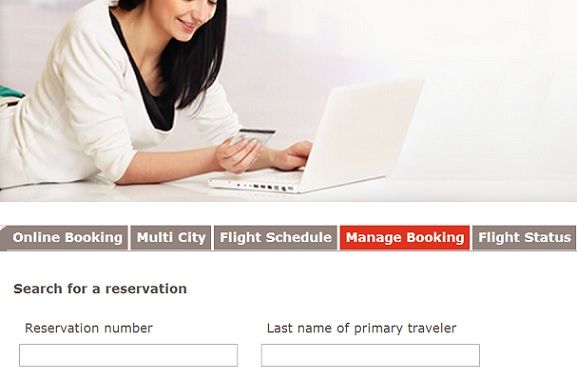A woman with long black hair cascading past her shoulders is photographed laying on her stomach, engrossed in her online activity. She wears a white long-sleeved shirt over a black top and is positioned with a laptop computer in front of her. With her left hand on the keyboard and her right hand holding a credit card, she appears to be finalizing an online transaction. The visible part of the image shows her from the waist up. Below her, a series of gray boxes labeled from left to right reads: "Online Booking," "Multi-City Flight Schedule," "Manage Booking," and "Flight Status." Notably, the "Manage Booking" box is highlighted in red. Further down, black text prompts the user to "Search for a Reservation," followed by another line containing smaller, less bold text stating "Reservation Number" with an accompanying text box beneath it. To the right, another prompt reads "Last Name of Primary Traveler," with a matching text box positioned below.